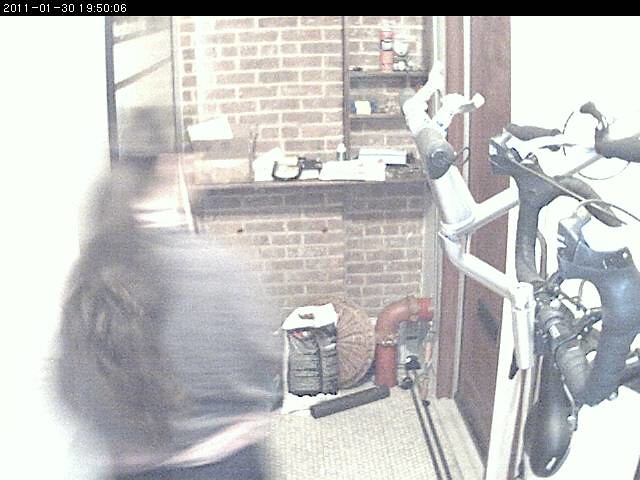The image appears to be a still from a CCTV camera dated 2011-01-30 at 19:50:06, capturing a scene in what looks like a garage or mechanic shop. On the right-hand side, a bike is hanging from a bike rack. The wall facing the camera is constructed of brown brick and is lined with shelves cluttered with various objects, including what appears to be a white teddy bear and possibly a can of WD-40. Below the shelves, there's a conspicuous red pipe, a bag, and a circular decorative item, with a rug on the floor. On the left side of the image, albeit blurry, there is a person mid-stride heading towards a wooden door equipped with a mail slot. The person has long brown hair tied in a ponytail that reaches above their waist, and is wearing a dark jacket with white at the top and bottom, a gray sweater layered over a white turtleneck, and dark-colored pants.